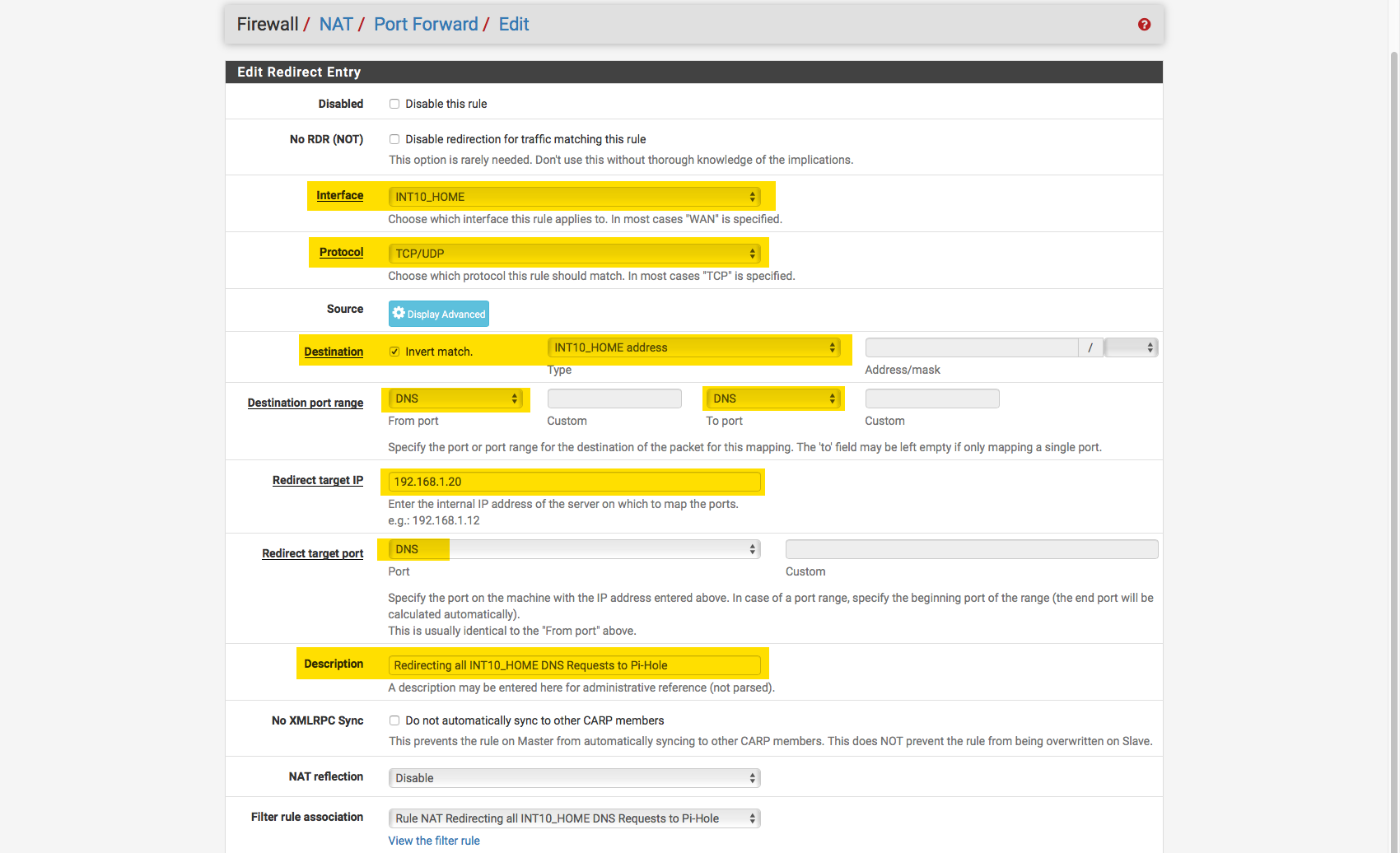Description of the Web Page Image:

The image depicts a web page interface for configuring a firewall rule. The page has a gray background and features a navigation bar at the top which reads "Firewall / NAT / Port Forward / Edit Firewall." In this navigation bar, "Firewall" is in black text, the slashes are orange, and the other words are blue.

Below the navigation bar is a section titled "Edit Redirect Entry." This section has a white background. The first option in this section is labeled "Disable this Rule," with a checkbox available to the right for disabling the rule. 

The following option is labeled "No RDR (Not)," with an empty bubble titled "Disabled redirection for traffic matching this rule." Beneath this, there is a note that reads, "This option is rarely needed; don't use this without thorough knowledge of the implications."

The next highlighted yellow section is labeled "Interface," and contains a drop-down menu titled "int10_home," which allows you to choose the interface to which the rule applies. A suggestion beneath this section notes that in most cases, "WAN" is specified.

Another highlighted yellow section labeled "Protocol" is present, offering a choice between "TCP/UDP." The advice provided suggests that in most cases, "TCP" is specified.

The "Source" section includes a blue "Display Advanced" button with a cog icon to its left.

In the "Destination" section, which is also highlighted in yellow, there is an "Invert Match" checkbox, a drop-down for "int10_home address," and a blank text entry bar followed by another drop-down bar.

The "Destination Port Range" section is next. It includes fields for specifying "DNS" in the "From port" field and provides an empty custom data entry bar. To the right is another custom empty field under the "To port" label with a note indicating that the port for the destination of the packet can be entered and that the "To" field may remain empty if mapping a single port.

The "Redirect Target IP" section is also highlighted in yellow, featuring a pre-filled text bar with the IP address "192.168.1.120." This represents the internal IP address of the server for port mapping.

The "Redirect Target Port" section contains a gray drop-down labeled "DNS" and an adjacent empty gray custom text box. A note beneath states that the port should match the machine with the specified IP address, and if dealing with a port range, the start port should be entered, while the end port will be calculated automatically.

Additionally, there's a yellow-highlighted "Description" section that reads "Redirecting all int10_home DNS requests to PH Ho." It notes that a description may be entered for administrative reference.

An underlined section labeled "No XML RPC Sync" includes an empty checkbox to the right with an explanation that this prevents the rule from automatically syncing to other members. The checkbox does not prevent the rule from being overwritten on the slave.

The "NAT Reflection" section contains a disabled drop-down menu.

Lastly, the "Filter Rule Association" section includes a drop-down menu that reads "Rule NAT Redirecting all int10_home DNS requests to PH Ho." Below this, in blue text, there is an option to "Review the Filter Rule."